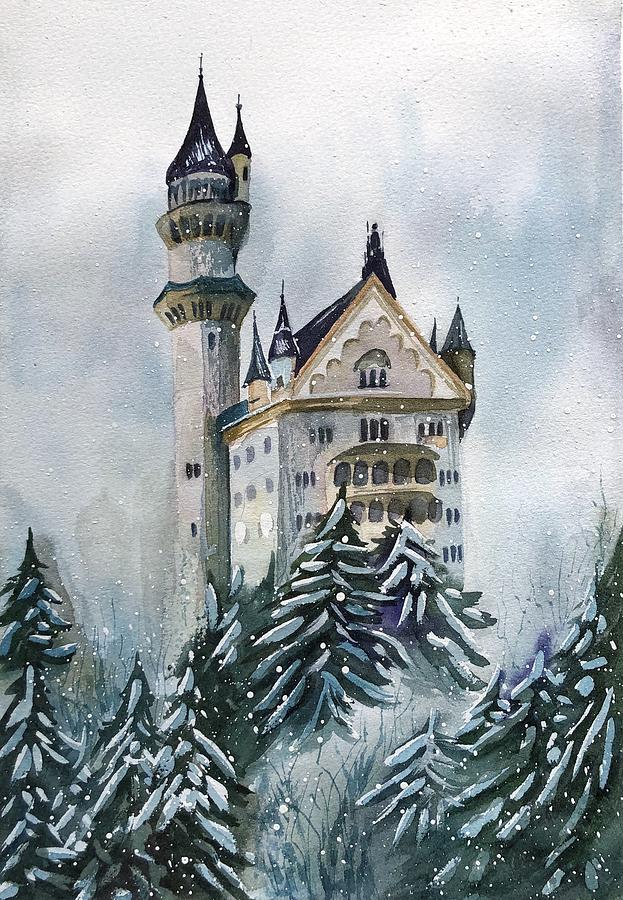This vertical rectangular artwork, possibly a painting or watercolor, depicts a wintry scene centered on a grand castle or large home, partially hidden by a dense assembly of pine trees. The sky, enveloping the upper sides and top of the scene, is textured with shades of gray and white, giving an impression of falling snow.

The primary structure in the middle is a predominantly white and brown castle or home, positioned on a hill and facing slightly to the right. The facade displays numerous windows and appears to have terraces. The pointed roofs peak from both sides, complemented by several steeples and conical structures. A prominent cylindrical tower with a rounded, pointed top rises significantly behind it to the left.

In the foreground, numerous dark green pine trees, dusted with snow, obscure parts of the castle. These trees are depicted with detailed white lines indicating snow on the branches. To the center bottom of the scene, there are thin green lines suggesting hints of grass or a pathway leading through the snow-blanketed landscape.

Overall, the artwork conveys a serene, snowy environment with intricate details of both the majestic structure and the encompassing frosty nature.